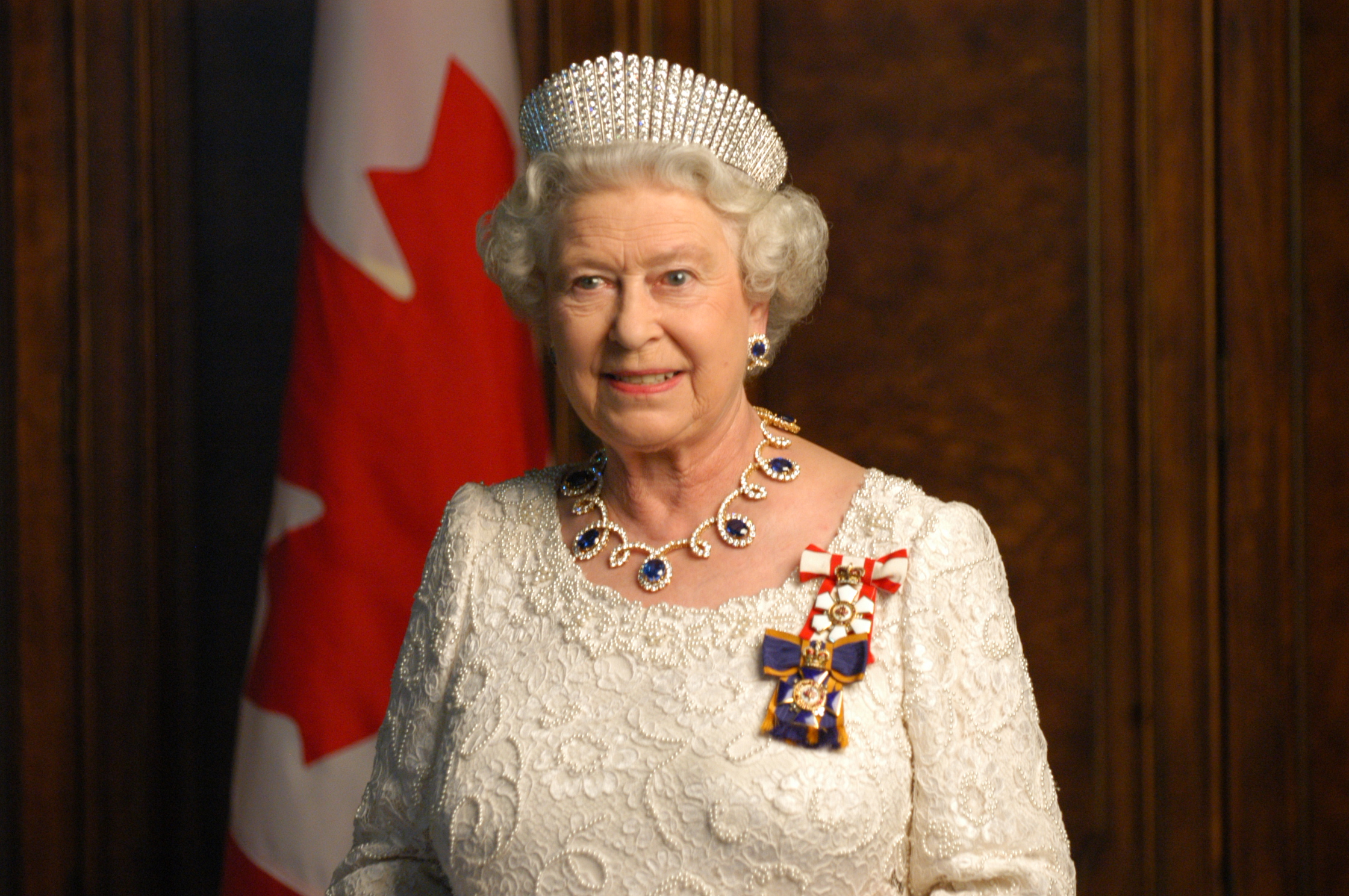In this detailed indoor portrait, Queen Elizabeth, adorned in a lace white dress, stands centrally against a brown wooden wall, partly illuminated by daylight. Her curly white hair is crowned with a diamond tiara that complements her blue earrings and intricate diamond necklace with a blue gem centerpiece, reflecting her regal splendor. She proudly wears a chest decoration featuring a red and white bow along with a blue ribbon, adding a touch of formality. The Queen's expression is a unique, gentle smile as she gazes slightly off-camera, her piercing blue eyes capturing attention. To her left, a red and white flag, likely the Canadian flag, hangs modestly, enhancing her authoritative yet approachable appearance. Adding to the visual harmony are accents of purple and gray amidst the dominant shades of brown, white, red, and blue. The photograph, free from any text, exudes a regal, historical ambiance, reminiscent of an image taken within a government building or formal chamber.